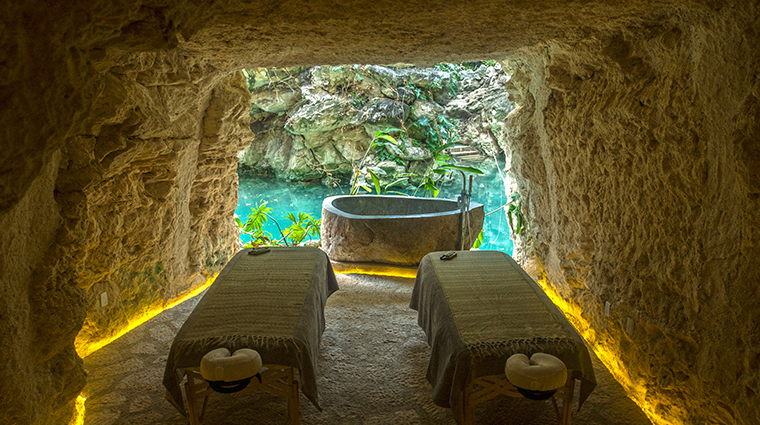The photograph, which appears to be taken at a luxurious spa retreat, captures the interior of a unique, square-walled brick cave with a low ceiling. The cave's walls, ceiling, and floor are constructed from brown and beige bricks, giving it a rustic yet elegant atmosphere. Inside the cave, the floor is paved with flagstone, and yellow perimeter floor lighting softly illuminates the space. Dominating the room are two massage tables, each draped with fringed coverings and equipped with headrests for face-down positioning during massages. Past the massage tables, the cave opens to reveal a serene view—tropical foliage surrounds a brick soaker tub filled with turquoise water, which seamlessly extends into a larger body of water. This calming aquatic scenery is framed by the cave's rock formations, enhancing the tranquil ambiance of the spa setting.